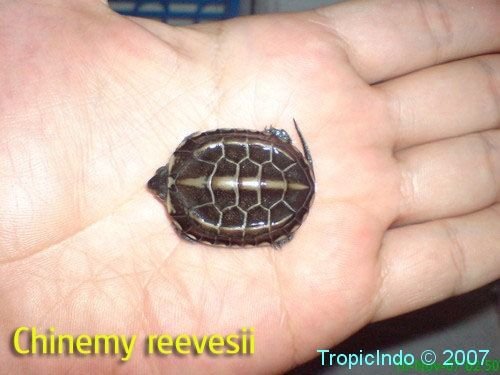This image, taken from above, captures a close-up view of a light-colored palm with the thumb stretched up and the fingers outstretched, holding a remarkably tiny turtle, roughly the size of a quarter. The turtle's dark brown shell features lighter spots and partially reveals its head facing left, along with its right back leg and tail peeking out slightly from the shell. The turtle's feet are mostly hidden. The bottom left corner of the image contains yellow text reading, "Chinamee Revesii," while the bottom right corner features light blue text that says, "Tropic Indo, © 2007."